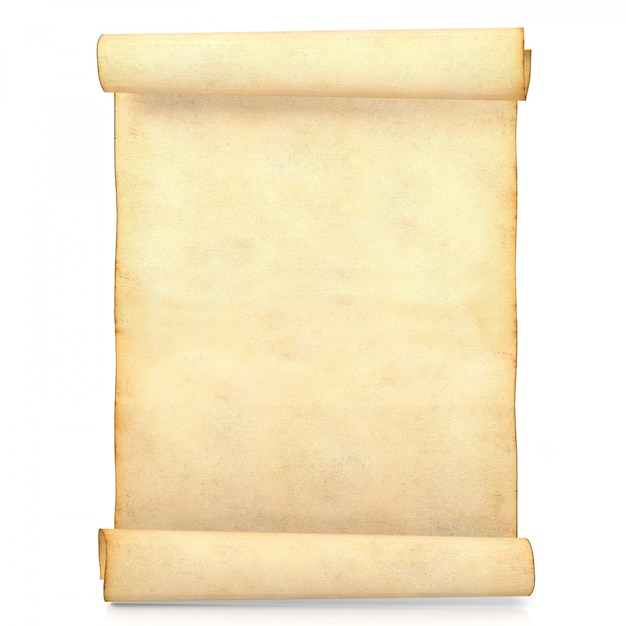The image depicts an aged, blank scroll set against a plain white background. The scroll, unfurled from the top and bottom, exhibits a yellowish, goldish hue with darker brown, crinkled edges, indicating its antiquity. The upper and lower parts of the scroll are rolled, giving it a characteristic scroll-like appearance. The paper's surface is bare, with no writing, drawings, or markings, and it shows subtle wrinkles suggesting a textured material, possibly parchment or a similar aged paper. The overall aesthetic, with its coffee-like tint and browned edges, emphasizes the scroll's vintage quality. There are no other elements present in the image—no people, animals, or objects—just the solitary, timeworn scroll.